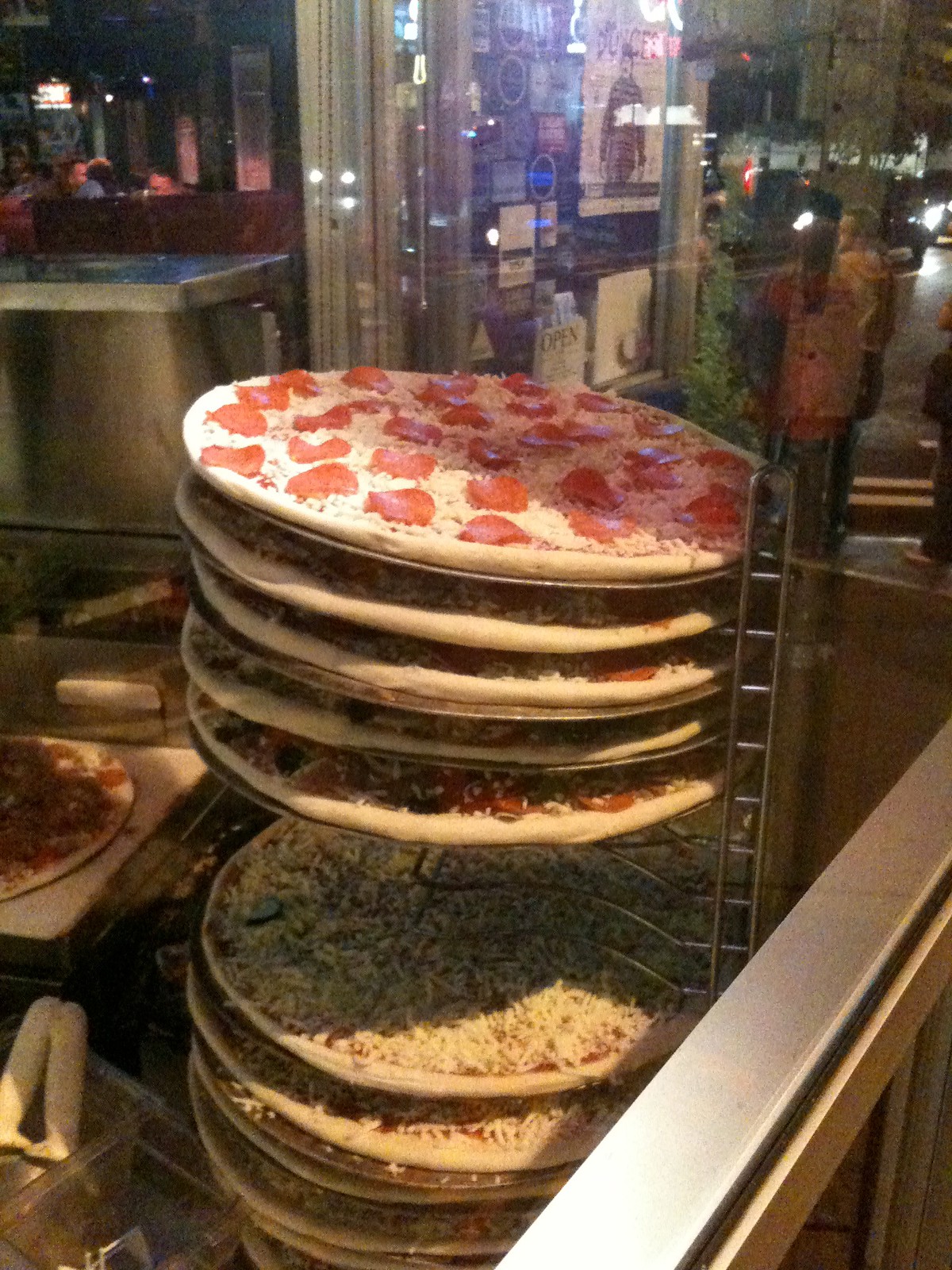The photograph captures the interior of a pizzeria at night, seen through a glass storefront window. Dominating the center of the image is a stainless steel wire rack brimming with uncooked, circular pizzas. At the top of the stack, a pizza adorned with pepperoni slices and scattered grated cheese sits in stark detail. Below it, several more stacked pizzas are visible, though their toppings remain indistinct due to the close arrangement. Noticeably, a gap in the racks reveals a solitary plain cheese pizza.

In the foreground to the left, part of a stainless steel kitchen countertop and miscellaneous kitchen equipment are visible. Ambient lighting conditions cast parts of the scene into shadow, particularly towards the bottom and lower left of the image. Moving up and to the right, the reflective glass reveals a blurred street scene with dark tarmac, double yellow road lines, and faint images of people outside, possibly glancing at wall posters. Beyond the street, a blurred view suggests cars with headlights on, signaling nighttime.

Further details in the background show various preparation items such as plastic buckets and utensils, hinting at the bustling activity of the pizzeria's kitchen. A high table with a thick surface, likely a worktop, is also discernable amidst the busyness. The image captures not just the preparation of food, but the lively environment of a working pizzeria with the promise of freshly baked goods soon to emerge from the oven.